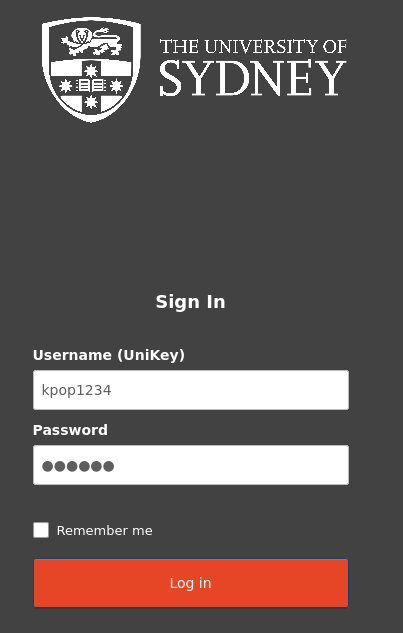This image is a screenshot of a login page for the University of Sydney's website. The background is solid black, with the university's name prominently displayed at the top in bold white text. To the left of the university name, there is a detailed logo resembling a shield that features elements such as armor, a tiger, four stars, and a black cross in the center.

Further down the image, there is a login section. Here, a text box labeled "Username" includes the placeholder text "Unikey" in parentheses, with the example username "kpop1234" already filled in. Beneath the username field is a second text box labeled "Password," positioned for the user to input their password. Below these fields is an option labeled "Remember Me," with a small white checkbox next to it.

At the bottom of the image, continuing with the black background, there is a prominent red action button labeled "Login," which invites the user to proceed with signing in.